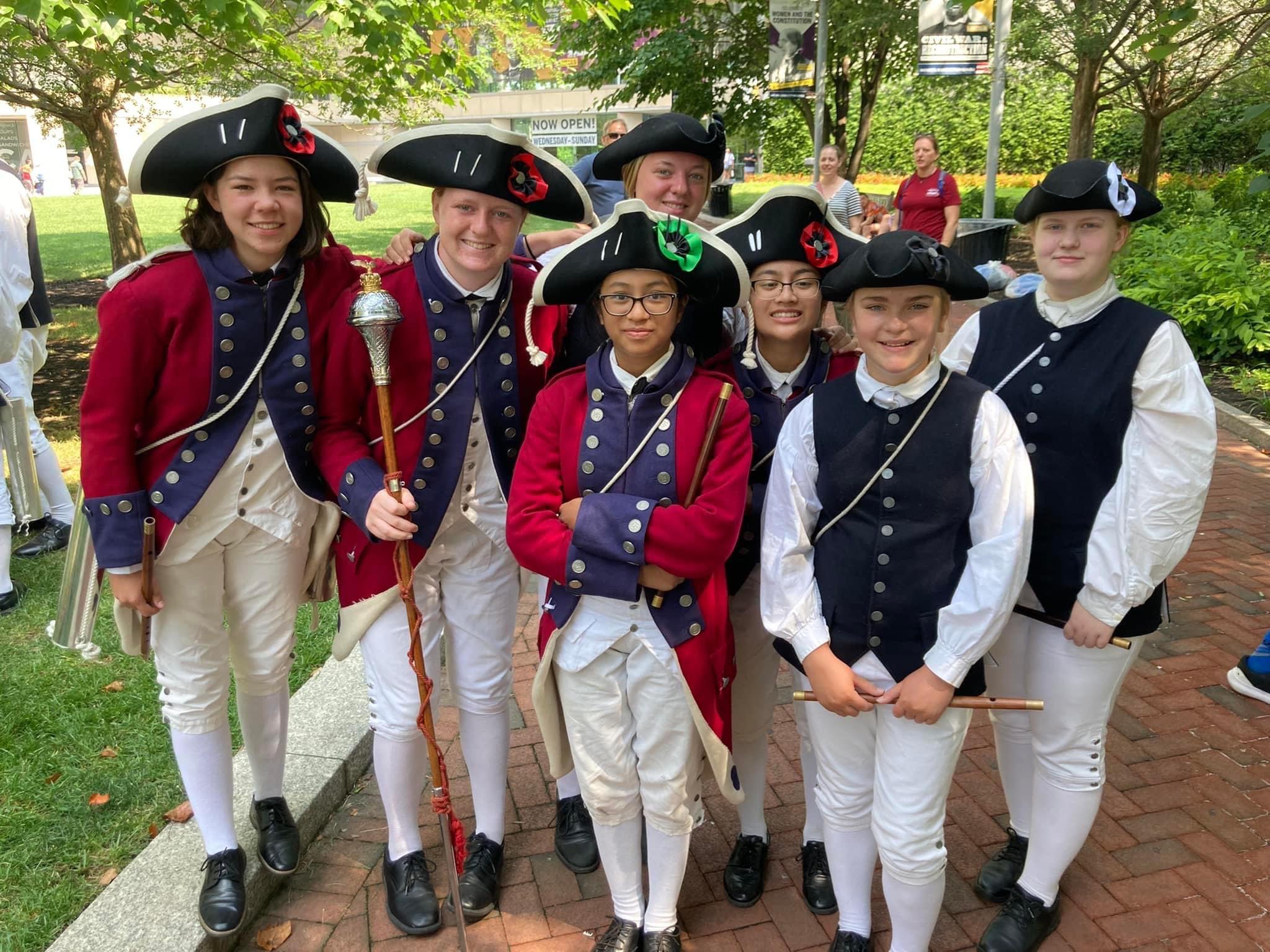In this vibrant color photograph, a group of seven children are intricately dressed as Revolutionary War re-enactors, striking a pose on a cobblestone pathway. All the kids sport distinct black hats, some adorned with red flowers. The group is divided in attire: three of the children wear striking red jackets that feature blue stripes down the middle, blue cuffs, and silver buttons, reminiscent of British soldiers. The remaining three are clad in blue vests with silver buttons over white collared shirts, mirroring the American Revolutionary Patriots. Additionally, one child on the second left holds a marching cane like a band leader, while two boys to the right are equipped with flutes, adding authenticity to their reenactment. Across the group, everyone is coordinated in white pants, long white socks, and black shoes.

The setting is an outdoor park bathed in sunlight, suggesting the photo was taken on a bright, pleasant day. Large rows of trees and patches of verdant grass frame the background, where a few other people stand. Behind the children, a building boasts a sign that reads, “Now Open Wednesday to Sunday.” The scene is further detailed with poles adorned with banners, adding to the historical ambiance. In essence, this image vividly captures the youthful energy and historical spirit of these young re-enactors against a picturesque outdoor backdrop.